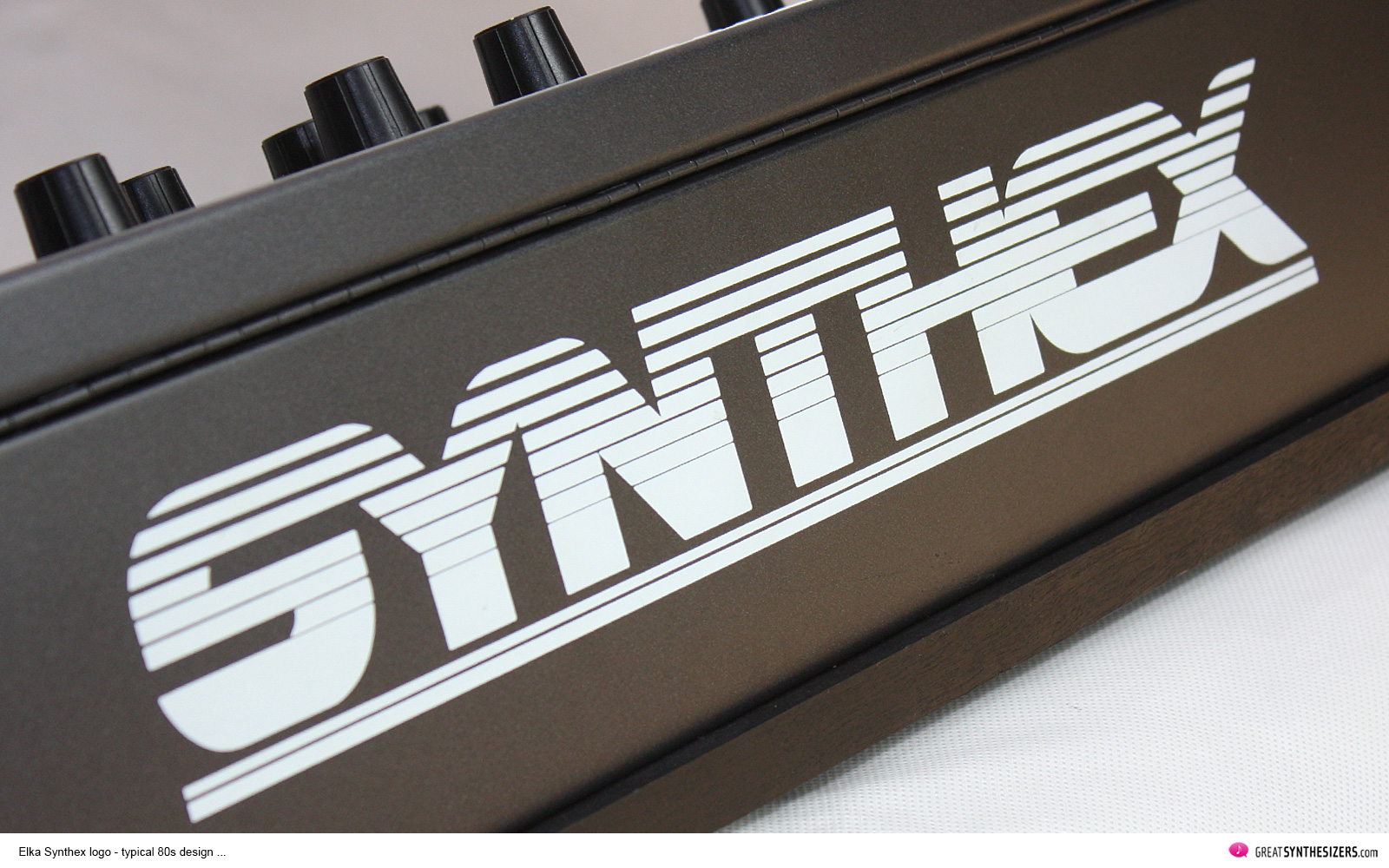This horizontal, rectangular black and white image showcases an electronic piece of equipment set against a grayish-white backdrop. The equipment itself is positioned diagonally across the picture, casting a shadow at the bottom. The object is black and bears the company logo "SYNTHEX" prominently in uppercase white letters indicative of a stylized font where the upper portions of the letters have black stripes. 

The surface of the electronic device features a variety of dark-colored circular caps—likely covering knobs or battery terminals—arranged in two rows. Visible in the image are five complete caps and the start of more. The setting appears well-illuminated, suggesting an indoor environment, with part of a clean white floor and a section of a beige wall subtly visible in the background.